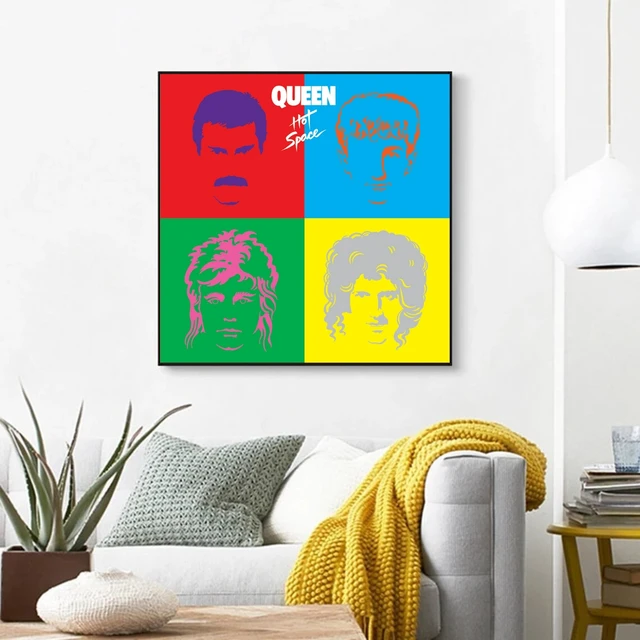This photo captures a modern, stylish living room with white walls that provide a neutral backdrop for the vibrant focal point—a pop art style poster of the band Queen. The poster prominently features the word "Queen" in white at the center top, with "Hot Sauce" written underneath. The design is segmented into four colored blocks arranged clockwise: red featuring a minimalist portrait of Freddie Mercury at the top left, blue with a portrait of the drummer at the top right, green with the other guitarist at the bottom left, and yellow with Brian May at the bottom right.

The room is furnished with a large pale gray sofa, accentuated by a white and gray throw pillow and a mustard-colored throw rug, giving it a cozy yet contemporary feel. In front of the sofa, a wooden coffee table holds a low, white cement vase containing a spiky cactus plant, adding a touch of greenery to the space. 

On the right side of the image, a hanging lamp descends from the ceiling, illuminating a round side table cluttered with books, magazines, and a glass of water, which all add to the lived-in charm of the room. This detailed and thoughtfully arranged living room combines elements of modern decor with personalized touches, creating an inviting and visually appealing space.